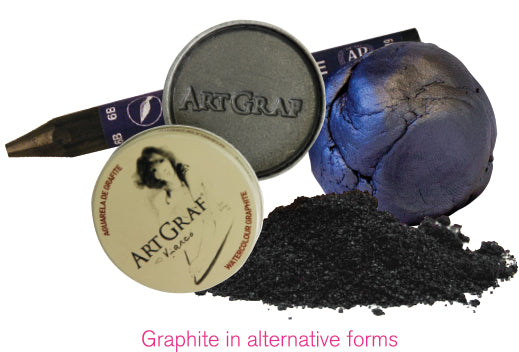The image presents a detailed advertisement for ArtGraph art supplies, showcasing graphite in alternative forms. At the bottom, printed in pink text against a white background, the image reads "graphite in alternative forms." Central to the composition is a tin container labeled "ArtGraph" in black text on a light beige background, which also features an illustration of a woman created using graphite. The open tin reveals solid black watercolor graphite. Surrounding the tin are various forms of graphite: a black powder, a dark silver-gray ball with visible fingerprint impressions, and a long graphite pencil marked "6B" with a partially obscured blue label, suggesting the versatility and creative potential of the product.